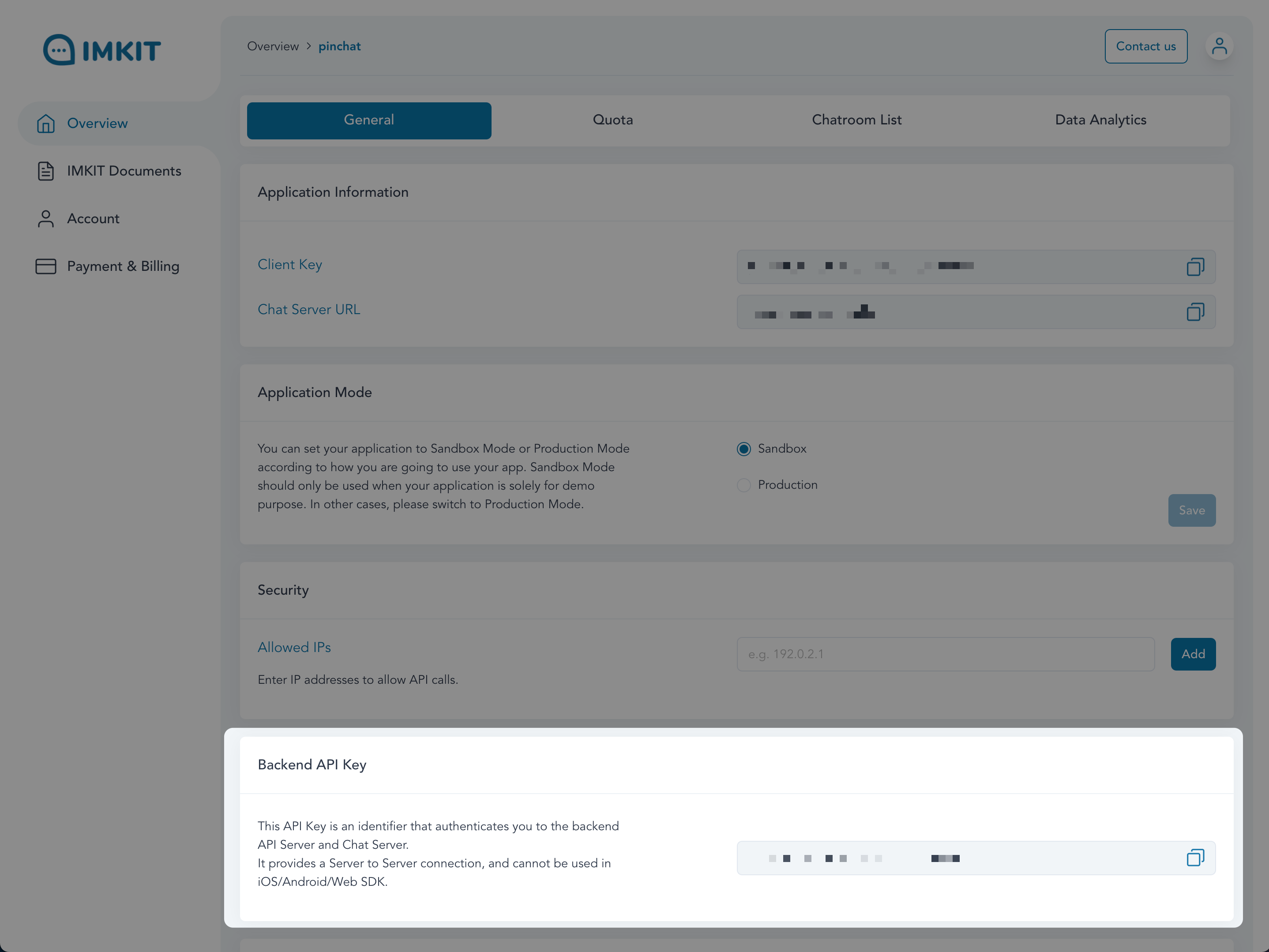This screenshot from the IMKIT website prominently displays the application's interface. In the top left corner, "IMKIT" is written in blue letters. Below this header are the navigation options: "Overview," "IMKIT Documents," "Account," and "Payment & Billing." The top of the interface features several tabs— "General" (highlighted in blue), "Quota," "Chatroom List," and "Data Analysis."

The central section contains application-specific details, including "Application Information," "Client Key," and "Chat Server URL," all of which are redacted. The application mode is set to "Sandbox," and there is an option for "Security" that facilitates various IP configurations, though these details are greyed out.

A prominent bright white panel overlays the bottom part of the screen. This panel, with black text, focuses on the "Backend API Key." The text explains: "This API key is an identifier that authenticates you to the backend API server and chat server. It provides a server-to-server connection and cannot be used by iOS, Android, or Web SDK." Blurred segments likely conceal the actual backend key.